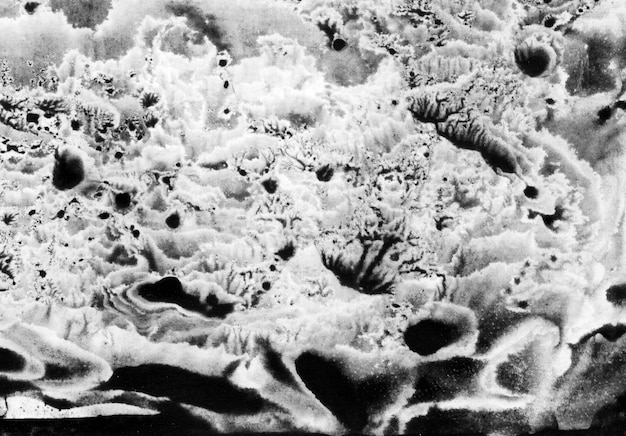This is a black and white microscopic image showcasing a series of irregular, holey structures. The shapes within the image are uneven and lack uniformity, indicative of a magnified view of an object or material at the cellular or sub-cellular level. The image is wider than it is tall, and it contains no discernible text, people, animals, plants, buildings, or vehicles. The intricate pattern of holes and the monochromatic tone suggest an abstract composition, emphasizing the complex and detailed nature of the subject matter.